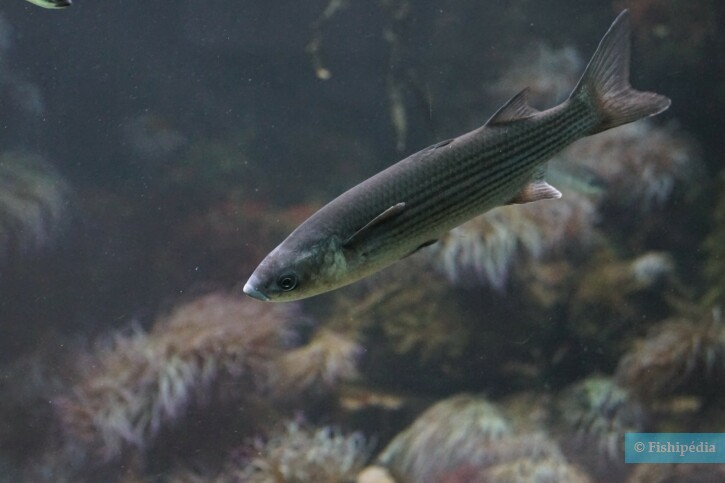This underwater photograph, likely taken in a lake, river, or possibly an aquarium, prominently features a lengthy, needle-pointy fish, swimming in the middle of the frame. The fish's coloring ranges from dark gray to blackish, with subtle blue-green hues on its head and faint striping along its body. Its dorsal and tail fins are discernible, suggesting an elegant, streamlined form. Although the overall setting is somewhat murky and dim, the background reveals glimpses of underwater plant life, possibly algae, coral, or anemones with long, leaf-like branches in brownish and white tones. Adding a touch of mystery and intrigue to the image, the bottom right corner contains a watermark with white text on a blue background that reads "Fishipedia."